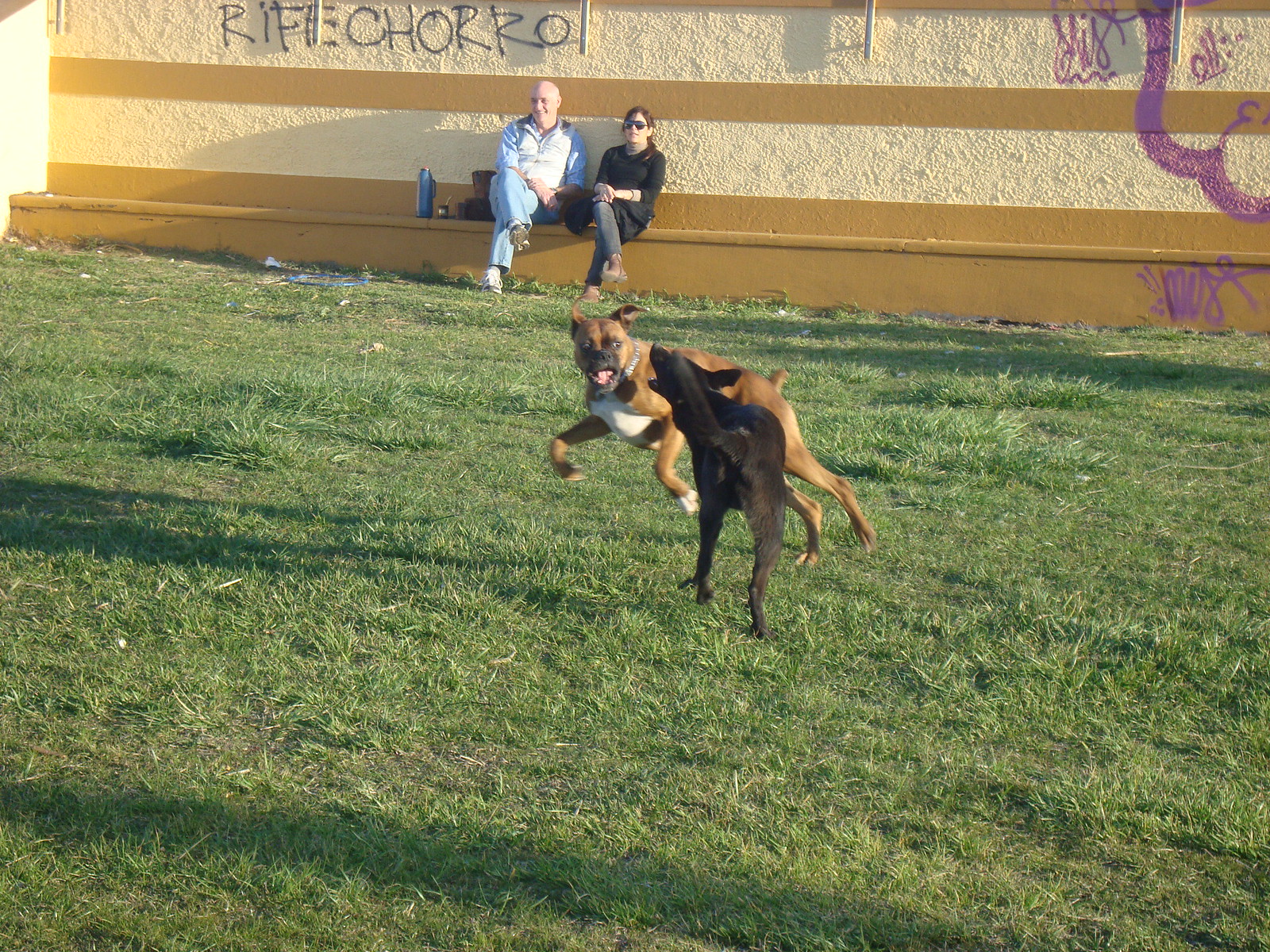In this image, a lively scene unfolds in what appears to be a dog park with a slightly overgrown grassy field. Two dogs, one resembling a Boxer and the other likely a black Labrador or possibly a German Shepherd, are energetically playing, seemingly chasing each other across the grass. In the background, two people, a man and a woman, are seated on a bench. The woman, dressed in a black top, black pants, and brown shoes, is wearing sunglasses, while the bald man dons a white jacket, jeans, and shoes. Behind them, graffiti is visible on a wall, prominently featuring purple shapes and writing with the phrase "R.I.F.E.C.H.O.R.R.O." There is some litter, including a water bottle near the seated man, scattered around their area.